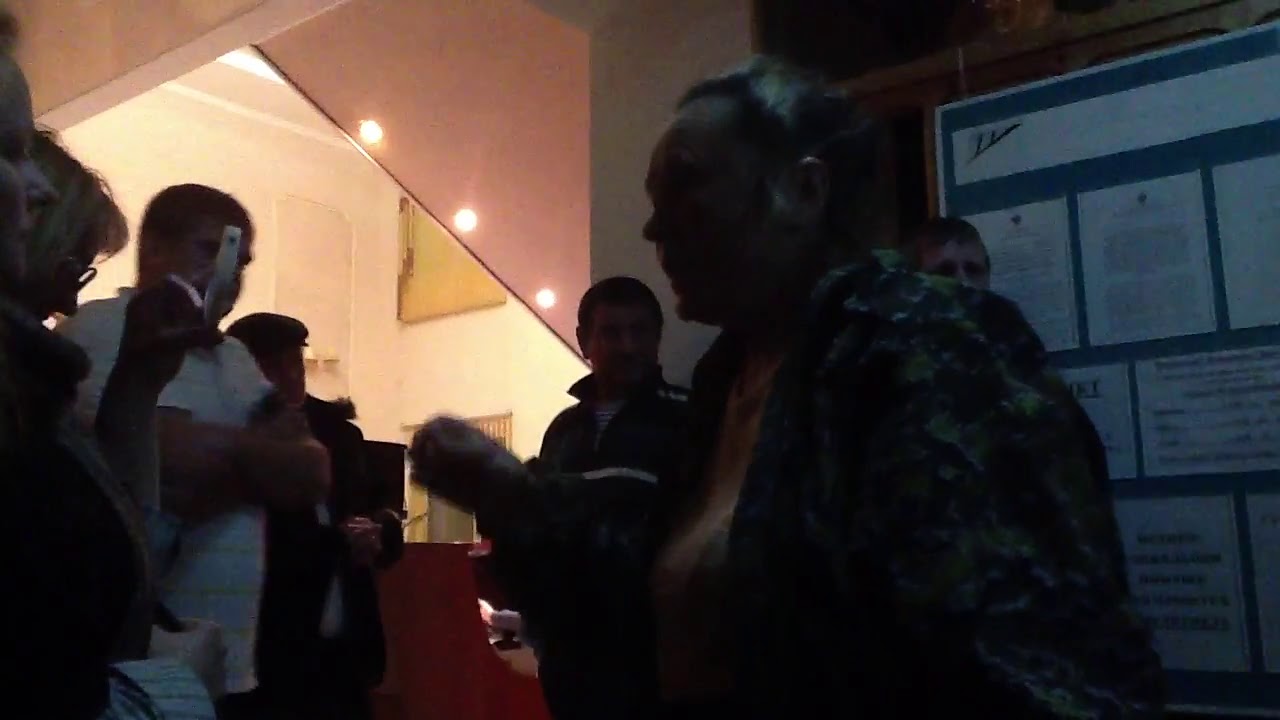The image captures an indoor scene featuring a group of people engaging in a conversation. At the center of the image, a woman is seen wearing a green and black sweatshirt over an orange shirt, standing in front of a bulletin board covered with several white pieces of paper bearing text. The scene includes both men and women who appear to be gathered casually in the room, with some of them possibly taking photos. One man in the group is distinguishable by his white shirt with yellow stripes. The right side of the image also features a blue poster board with additional papers tacked onto it. In the background, a white wall with a portrait hanging on it and a hanging pink fixture with multiple lights can be observed. The overall lighting is dim, but there are several lights turned on in the room, illuminating the scene. The colors in the image range from white and black to blue and green.